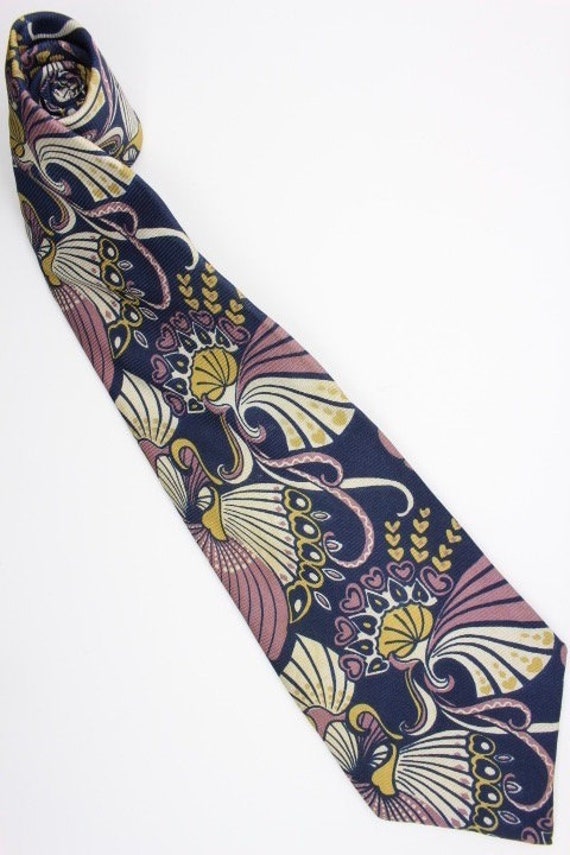This is a detailed photograph of a man's necktie, captured against a pristine white background. The necktie is partially rolled up at the narrow end, which occupies the top left of the image, while the broader, unrolled section extends diagonally toward the bottom right corner. The high-quality tie, made of silk, showcases a dark blue to purple backdrop adorned with large, abstract, tropical floral designs that include shades of yellow, purple, and white. These intricate patterns evoke the appearance of fancy tropical wallpaper, with elements resembling swirling shapes and fan-like motifs, giving the tie an elegant, luxurious look.